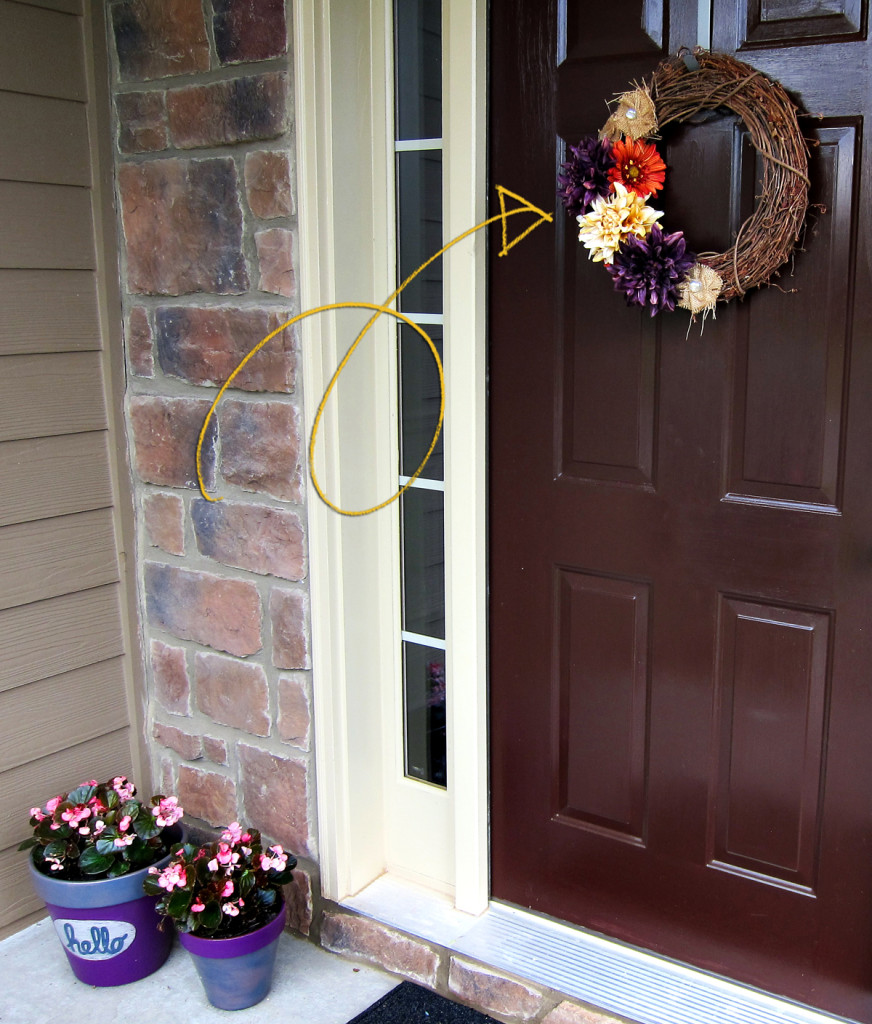The photograph captures a charming entrance of a house featuring a large brown door situated centrally in the image. Adorning the door is a decorative wreath showcasing an array of colors: brown, red, purple, white, and tan. Above the door, a piece of gold-colored rope forms an arrow pointing towards the wreath. Adjacent to the door on the left is a small side window framed in white, enhancing the inviting appeal of the entryway. The left portion of the image reveals a red and gray brick wall, adding a rustic touch to the setting.

At the base of the image, in the bottom left corner, two vibrant potted plants can be seen. The plant holders, colored in shades of purple and blue, have green and pinkish-red plants sprouting from them. One of the plant holders bears the word “Hello” written in cursive, further indicating a warm welcome. The scene is grounded by a black welcome mat, highlighting the transitional space from outside to inside. Overall, the photograph exudes a warm, homely feeling, perfectly capturing an inviting front entrance of a house.